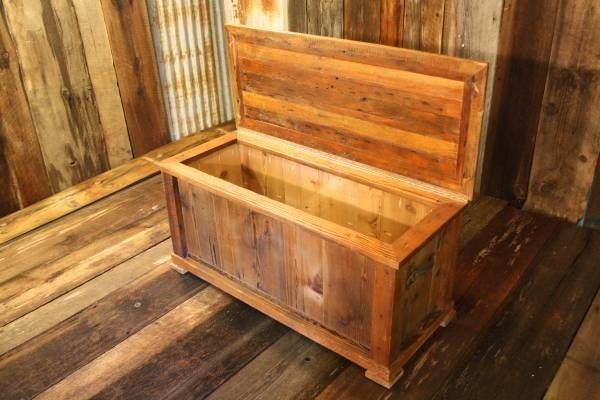This image features a well-crafted medium-sized cedar chest with an open lid, situated in a room where everything is made of wood. The floor consists of wooden planks and the walls are also paneled in wood, giving the room a sauna-like appearance. The chest, designed to protect clothing—especially wool sweaters—from moth damage, appears very sturdy with precise wood fittings at the corners. It has small square feet providing a slight elevation, and there is some illegible writing on the side. The meticulously constructed woodwork includes an indentation on the underside of the lid, ensuring a secure closure.